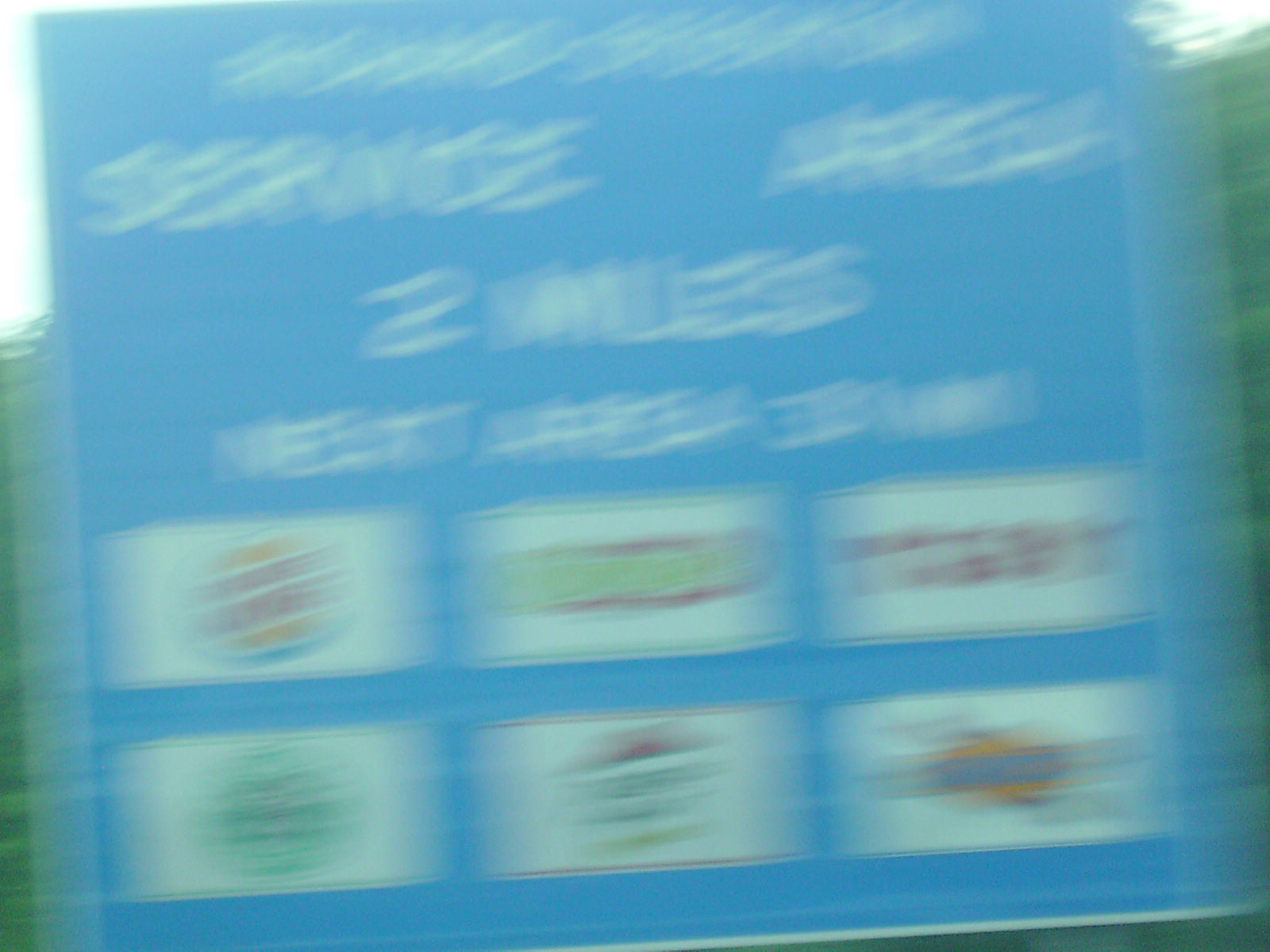The photograph depicts a blurry blue road sign indicating a service area 2 miles ahead, accompanied by six logos for various services and eateries on a white background. Arranged in two rows of three logos each, the top row features Burger King on the left, a Blimpie sandwich shop in the middle, and a logo with red lettering on the right that is hard to identify. The bottom row includes Starbucks on the left, Pizza Hut in the middle, and an indiscernible logo with some orange detail on the right. The background shows some greenery, suggesting a forested area. This sign typically aims to inform travelers of available amenities to help them decide if they need to stop for gas, food, or other services, making it a useful planning tool for those on the road.